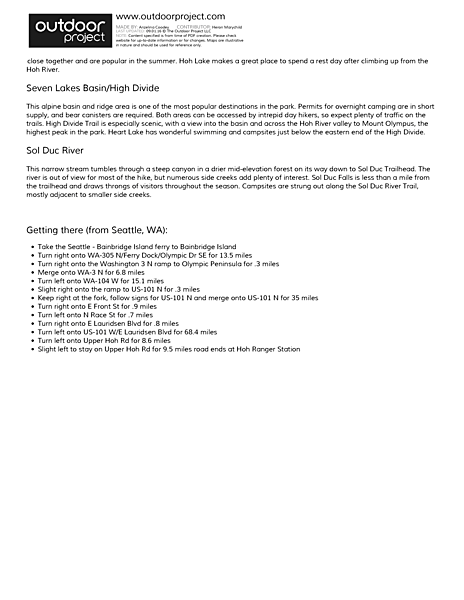In the upper left corner of the image, the "Outdoor Project" logo is prominently displayed within a black rectangle, featuring white text. Below the main text, there is small, illegible writing due to poor resolution.

The caption reads:

"Hop Lake is an ideal spot to relax after ascending from the Hoh River. The Seven Lakes Basin area, including the High Divide ridge, is one of the most popular destinations in the park. During summer, the trails and camping sites see heavy traffic, and permits for overnight camping are scarce. Bear canisters are mandatory for campers. Although challenging, the area is accessible to determined day hikers, often leading to busy trails. The High Divide trail offers particularly scenic views into the basin, across the Hoh River Valley, and towards Mount Olympus, the park's highest peak. Hart Lake is also notable, with excellent swimming opportunities and campsites located just below the eastern end of High Divide. Additionally, the Sol Duc River is mentioned."